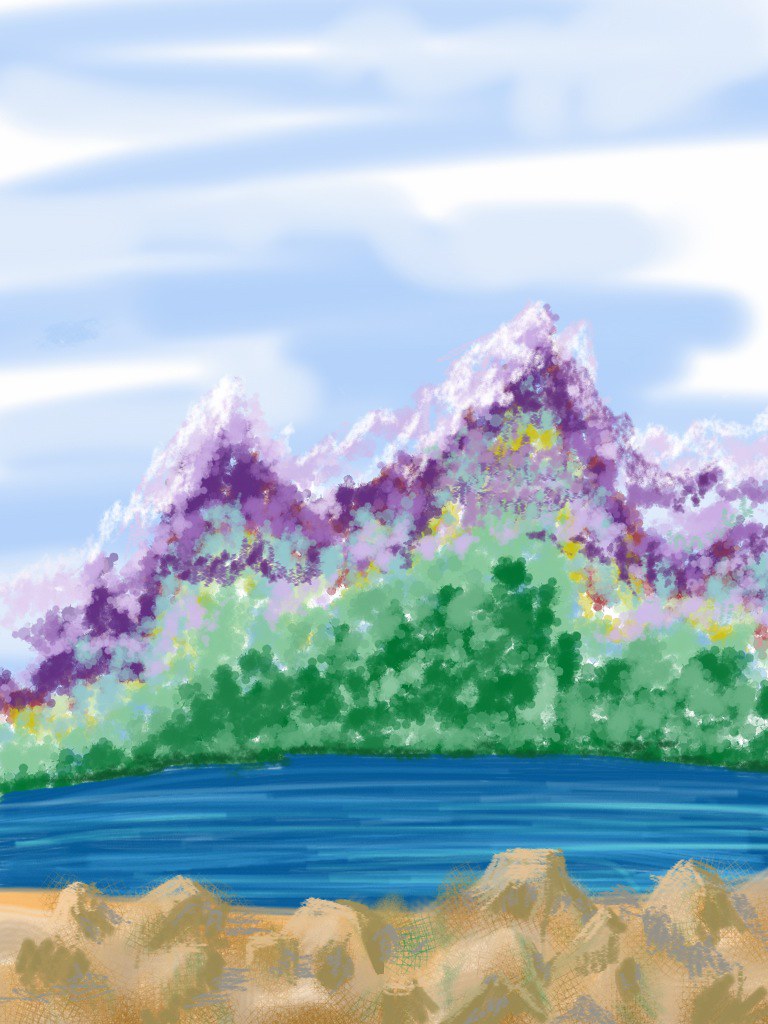In this intricately painted image, the foreground features a rocky surface composed of tan and brown hues, meticulously rendered to evoke the texture and form of natural rocks. Above this rugged terrain lies a body of water, depicted with varying shades of blue that streak horizontally across the canvas, capturing the fluid motion and reflective quality of water. Rising above, splotches of green paint ascend into a towering peak, transitioning into lighter green tones as the ascent progresses. The summit is adorned with a blend of purple and white, skillfully applied with a paintbrush to simulate the snow-capped apex of a mountain. The sky dominates the upper portion of the image, characterized by dynamic, slashing brushstrokes in shades of blue and white, suggesting a vibrant, yet serene atmosphere. The overall composition harmoniously combines the rugged earth, tranquil water, majestic peaks, and expansive sky, creating a captivating and detailed work of art.